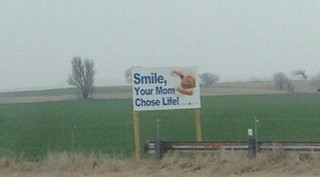In this small, low-resolution, horizontally oriented snapshot, a pro-life advertisement is prominently displayed in a rural, possibly Midwestern landscape. The photograph is taken outdoors, on a seemingly overcast and muggy day with a completely gray sky, hinting at smog. The image captures a wide, flat, green field stretching across the foreground, edged by some dark brown brush, and dotted with sparse trees indicating a late fall or winter season. The focal point is a white sign with blue text declaring, "Smile, Your Mom Chose Life," accompanied by an image of a newborn baby wrapped in a white blanket. This sign is supported by two wooden poles and stands near a metal fence that runs along the bottom of the image, separating the overgrown grass from a patch of dirt. The overall scene conveys a subtle yet proud pro-life message amidst the quiet, desolate backdrop.